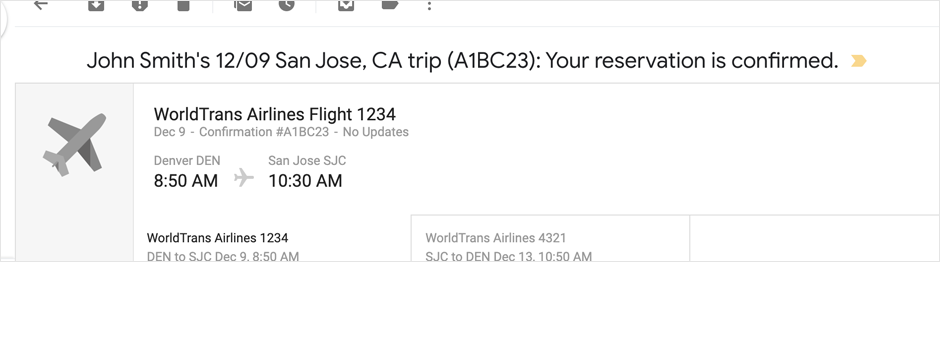This image is a cropped screenshot of an email confirmation for a flight booking. At the very top of the page, partial icons are visible on the top left, including an arrow pointing to the left, a save icon, an exclamation point within an octagon, a trash icon, an envelope icon, and a clock icon. 

In the main body of the email, there is a header that reads: "John Smith's 1209 San Jose, California trip" with numbers in parentheses following the text. Directly below, it confirms "Your reservation is confirmed."

To the left side, a gray panel features a thumbnail image of an airplane. Adjacent to this, on a white background, are the flight details. In the top left section of this area, it says "World Trans Airlines flight 1234," followed by the date and a confirmation status indicating "No updates." 

Further down, the departure airport and time are stated, accompanied by an airplane icon in the center pointing to the right, indicating the direction of the flight. Below this, the return date or destination is provided. Additional details about the airlines are present but unfortunately cut off or cropped out of the screenshot.